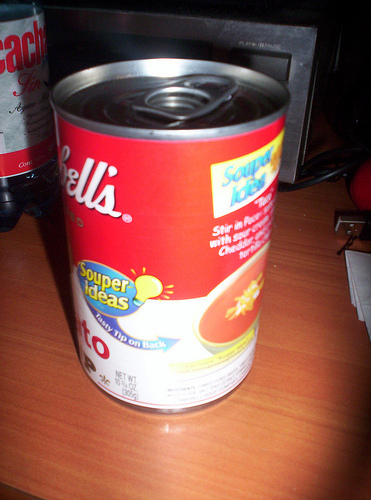A detailed side view photograph showcasing a can of Campbell's Tomato Soup prominently displayed at the center of a two-toned brown and tan table. The iconic Campbell's logo is partially visible, displaying "B-E-L-L apostrophe S," with the text "super ideas" and a yellow light bulb graphic underneath. This graphic features an arrow pointing downward toward a bowl of soup labeled "tasty tip on back." The can’s label reveals parts of the words "TOMATO" and "SOUP" with the letters "A-T-O" in red and the letter "P" in gold. The back of the can provides further details with the words "super ideas" in white lettering and an image of a soup bowl topped with what seems to be cheese. The top of the can is outfitted with a silver pull tab. In the background, there is an indistinct packaged product, possibly a soda bottle, on the left side. Additionally, there appears to be a microwave or another electrical appliance, along with a piece of paper, on the right side of the composition.